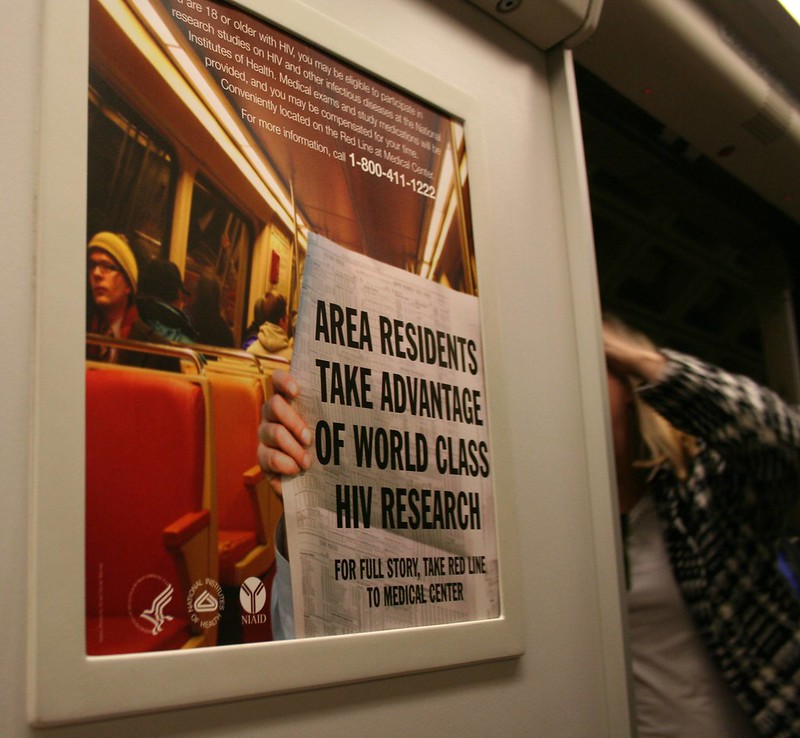This image depicts an advertisement poster hanging on a white wall, seemingly located inside a subway car. The poster portrays a scene within a subway car featuring passengers seated on red benches. Among them, one person in the lower right-hand corner is holding up a newspaper that prominently displays black blocky text stating, "Area residents take advantage of world-class HIV research." Below this, in smaller font, it instructs, "For full story, take the red line to Medical Center."

Above the newspaper, there's white overlay text informing, "If you are 18 or older with HIV, you may be eligible to participate in research studies on HIV and other infectious diseases." It provides a phone number for more information: 1-800-411-1222. The poster is further detailed with light strips that emit an amber-yellow glow, enhancing the ambiance of the subway car interior. It also includes health organization logos, reinforcing the advertisement’s focus on promoting awareness and participation in HIV research studies.